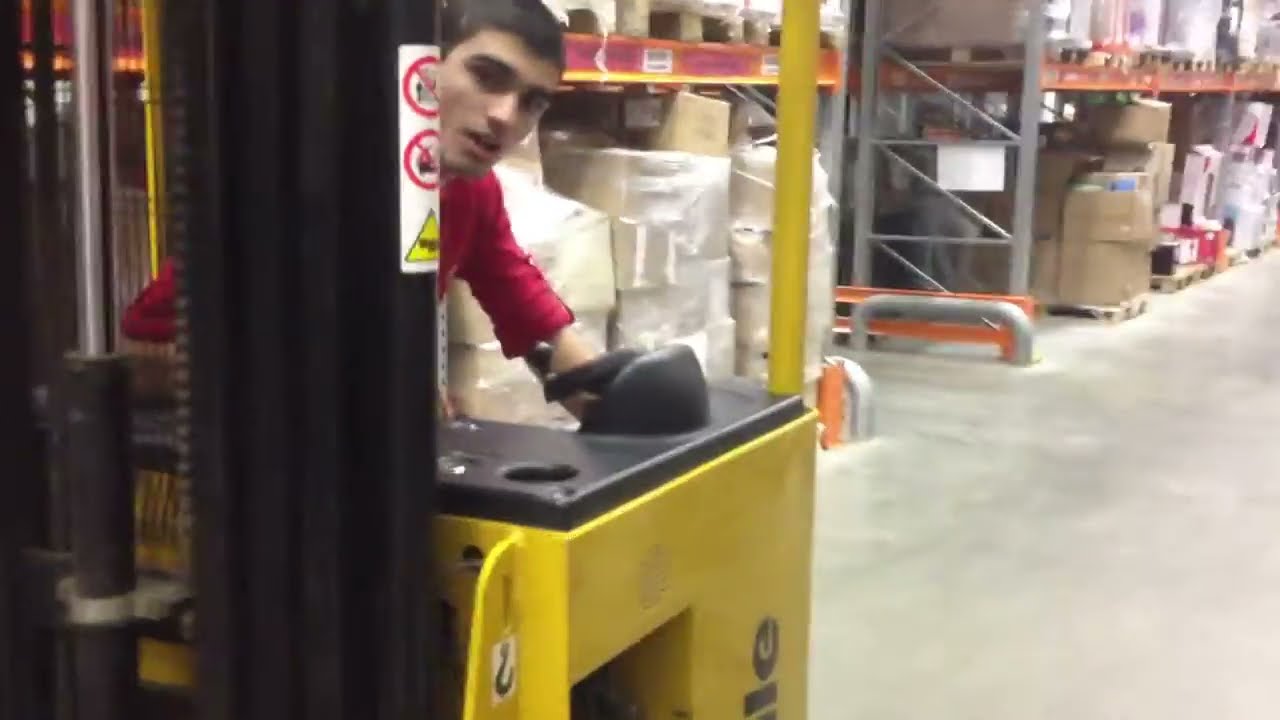In the image, a young man with dark hair, dark eyes, and dark eyebrows wearing a red shirt is driving a yellow and black forklift in a warehouse setting. The warehouse features stone-colored concrete floors and reddish-orange metal shelves filled with bulk items, mainly brown boxes wrapped in plastic or saran wrap. The man, who appears to be talking with his mouth slightly open, is leaning forward and staring directly at the camera from the forklift. The shelves and the floor underneath are packed with pallets and containers, indicating that this area might be a shipping station or an Amazon warehouse-type facility where packages are stored before being shipped. On the right side of the image, there is a distinct steel bumper area near an exit to prevent the forklift from hitting the doorway. The setting resembles a large back room of a store, similar to a Home Depot, with orange walkway highlights adding to the mix of industrial features.